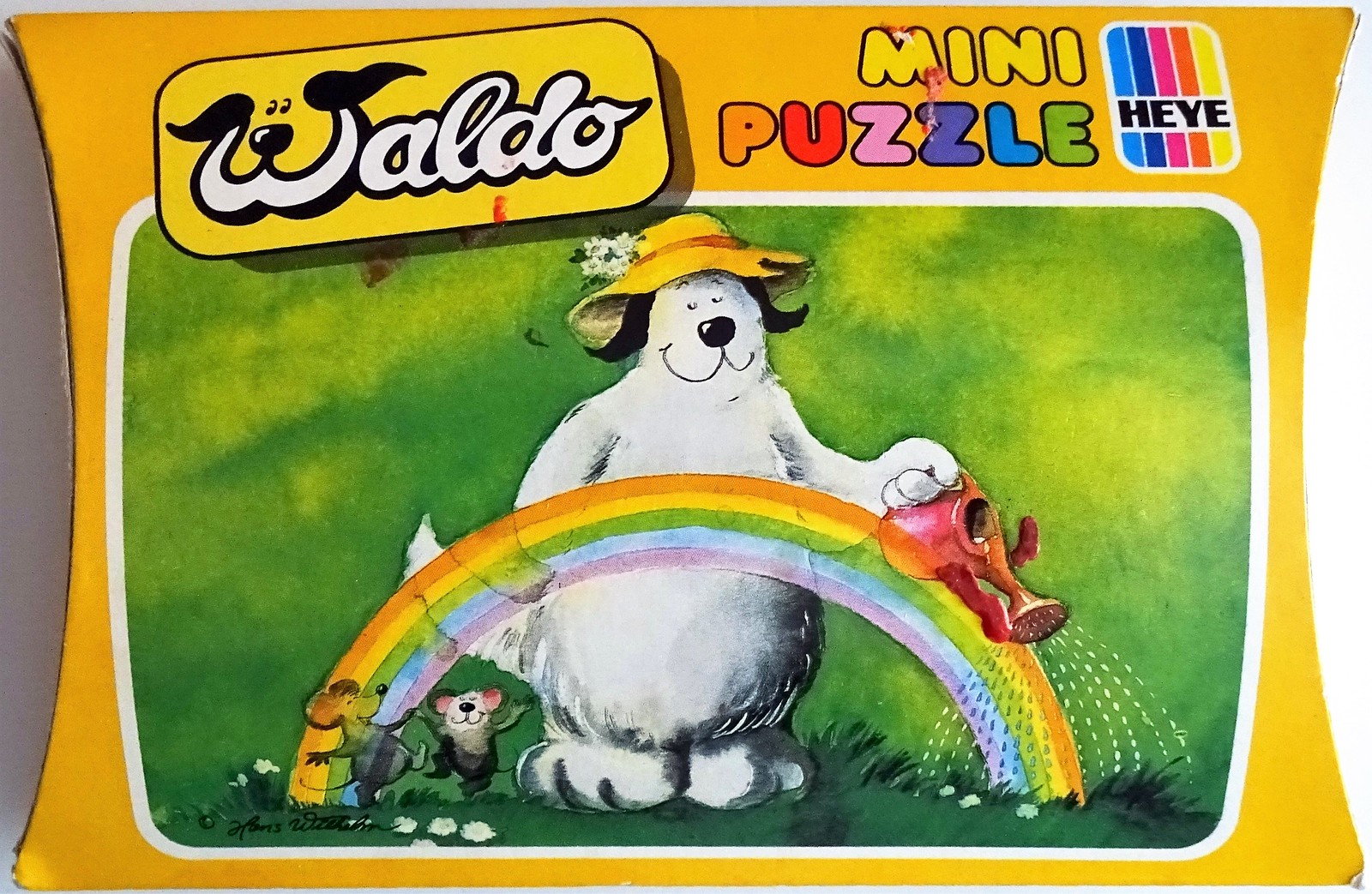The image depicts the cover of a puzzle box characterized by its striking dark yellow or orange theme. In the upper left corner, a yellow rounded rectangle with a blue border prominently displays the word "Waldo" in white letters. The "W" ingeniously forms the visage of a dog, with the two prongs resembling ears, eyes between them, and a nose at their intersection. Adjacent to this, on the top right corner, "Mini Puzzle" is written, with "Mini" in yellow and "Puzzle" in multi-colored letters: an orange P, red U, pink Z, purple Z, blue L, and green E. Next to these words is the vertical, rainbow-styled HE-Y logo with the word "hey" in black. The main artwork on the box features a whimsical white dog, identifiable from some descriptions as a polar bear, with a black nose and black hair. This character is adorned with a yellow hat, accented with a red ribbon and a white flower, standing on its hind legs while pouring water from a red watering can onto green grass. Behind this endearing figure is a vividly colored rainbow, and beneath, two gray and white mice are seen dancing joyfully. This charming and intricate design suggests that the puzzle is intended for children.